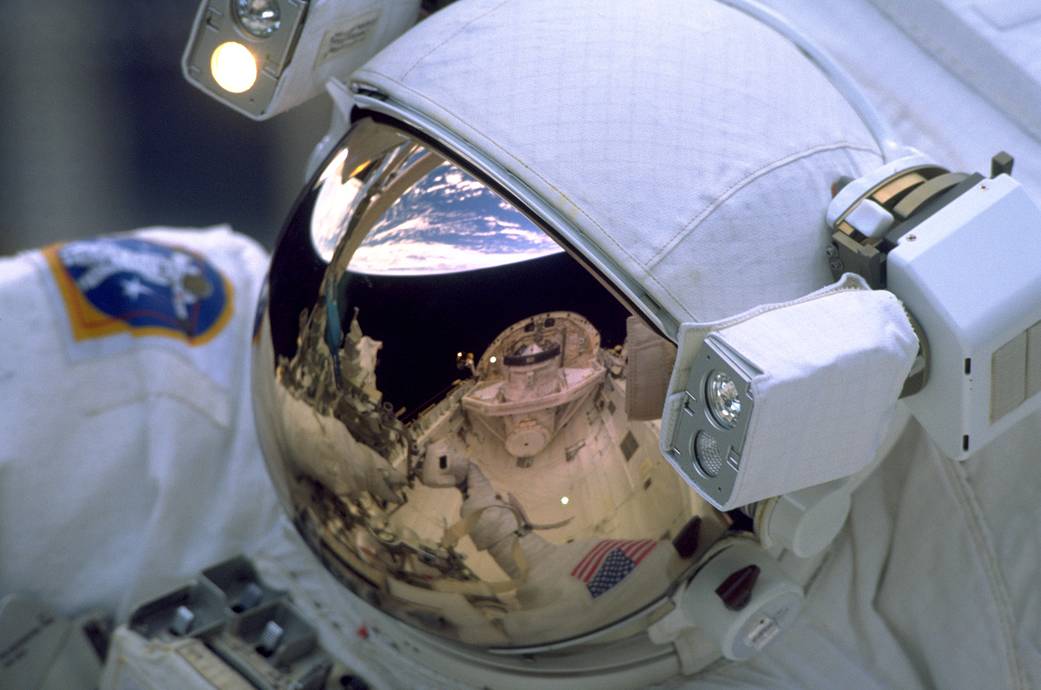In the forefront of the image is an astronaut in a white space suit, with a helmet featuring a mirrored visor that reflects the surroundings. On the right arm of the astronaut, there’s a prominent American flag patch. The helmet is equipped with a white cloth around the visor and a built-in light, which is illuminated, along with another light that is not turned on. The reflective visor displays a faint, upside-down image of an American flag, the Earth in the background, and possibly a portion of a space station or spacecraft. The blurred grayish backdrop adds an element of depth to the scene, emphasizing the distance and vastness of space, while the suit, identifiable up to the chest area, showcases intricate details with blue and yellow markings near the left side.